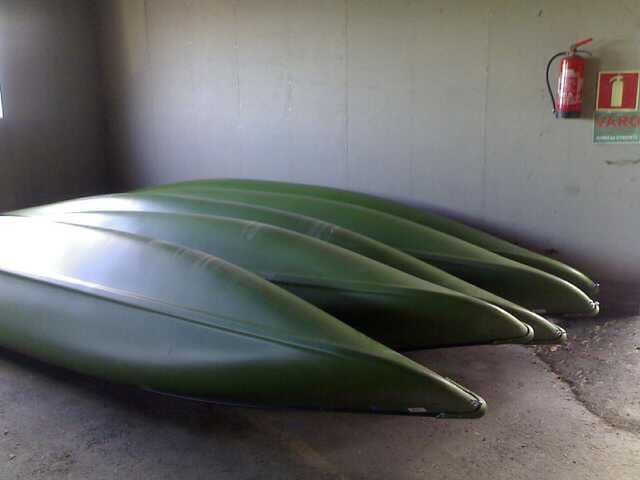This photograph shows five bright green canoes with their bottoms up, stacked and leaning against each other in a corner of a concrete garage. The garage floor and walls are made entirely of concrete, except for a small, barely visible window on the left side that allows some natural light to pour in. Additional light comes from a source on the right, which is of a different color. In the upper right corner of the image, a mounted red fire extinguisher is visible on the wall, flanked by two pieces of paper: a small red square with a white fire extinguisher silhouette and a larger green one with red lettering, the text of which is unreadable. The canoes' vibrant green color and smooth, clean surfaces give them a leaf-like or sideways banana appearance.